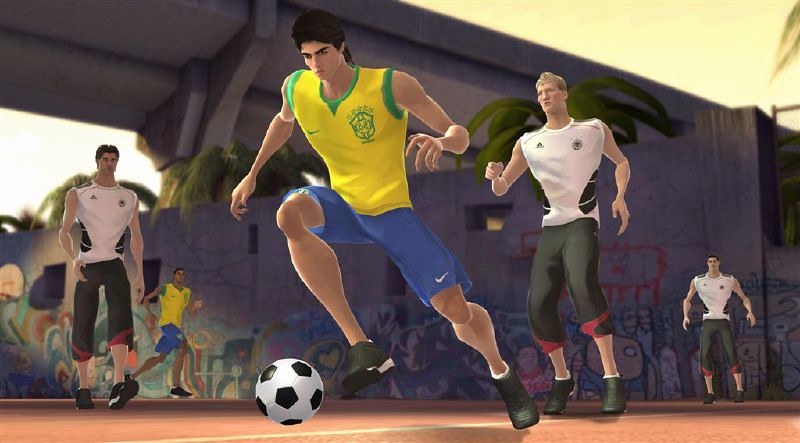This detailed and cleaned-up description provides a clear visualization of the digital image:

"In this vibrant digital image, which is almost twice as wide as it is high, we are immersed in the dynamic action of a street soccer match, possibly rendered from a video game. At the forefront, a group of four to five soccer players commands attention. Central to the scene is the prominent player in mid-dribble. His imposing figure spans nearly the entire height of the image, leaning slightly with his head tilted to the left. His right leg, bent at the knee, juts forward with the thigh nearly horizontal, while his left leg trails behind, semi-bent at the knee.

Dressed in long, medium-blue pants adorned with a small white Nike logo on the bottom-left pant leg, he also sports black shoes with only thin white socks visible above them. The classic white soccer ball with black patches hovers near his elevated right foot, merely inches off the ground, while his left foot appears to maintain light contact with the playing surface. His arms, partially extended with the left arm bent more than the right, suggest a poised yet agile stance. His gaze is intensely focused on the ball below, framed by thick black eyebrows and short black hair, adding to the overall intensity. Notably, his head appears disproportionally small compared to his broad chest and shoulders.

Adjacent to him on the right stands an opponent, who appears slightly upright with a vigilant stance. This player dons long, dark gray charcoal pants below the knees, complemented by black shoes and a sleeveless white shirt marked with black accents. His blond hair and similar robust body structure mirror those of the central player. Behind him, another teammate can be seen in the lower right corner of the image, sporting the same charcoal uniform, while another player, similarly attired, is visible even further back to the left.

The image's background portrays a street setting, characterized by a brownish-colored surface and surrounding walls covered in graffiti. Far behind the central action, on the lower left side, another player in a yellow shirt with green trim, matching the featured dribbler, is barely discernible. The image overall encapsulates the raw energy and street spirit of a soccer game."